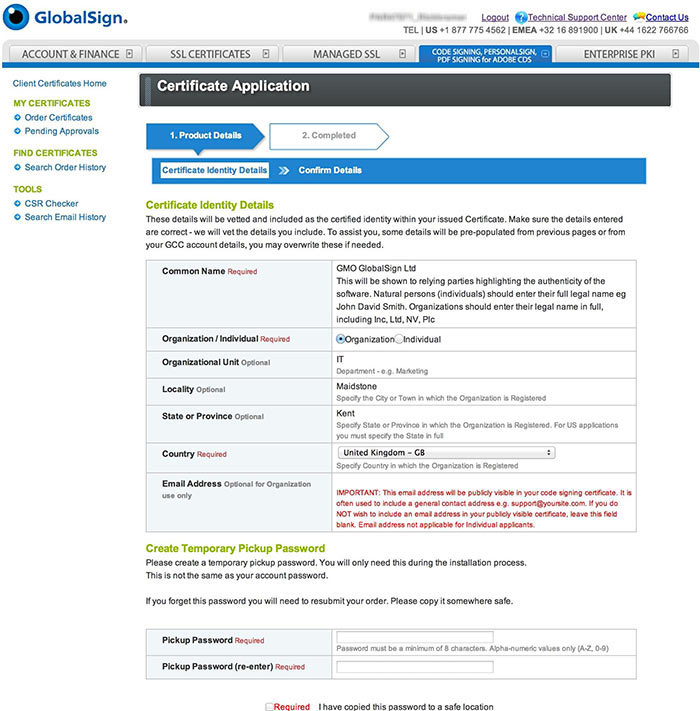This screenshot from a website features a predominantly white background. In the top left corner, the text "Global Sign" is displayed in blue next to a tealish blue circle with a black center, resembling an eyeball or camera lens, complete with a white reflection on the left side. The top right corner includes links for "Logout," "Technical Information," and "Contact Us," as well as telephone numbers in black font for the US, EMEA, and the UK.

Running horizontally across the top are menu tabs in an off-white color with gray font. The active tab is highlighted in a darker blue and reads "Code Signing, Personalization, PDF Signing for Adobe CDS." The inactive tabs, in light gray, are labeled "Account and Finance," "SSL," "Certifications," "Managed SSL," and "Enterprise PK."

Below the tabs, there is detailed content displaying product deals and certification details. This section includes a form with fields for "Common Name," "Locality," "State or Province," "Country," and "Email Address." There is also a "Pickup Password" section, suggesting functionality for collecting an item or accessing a specific service.